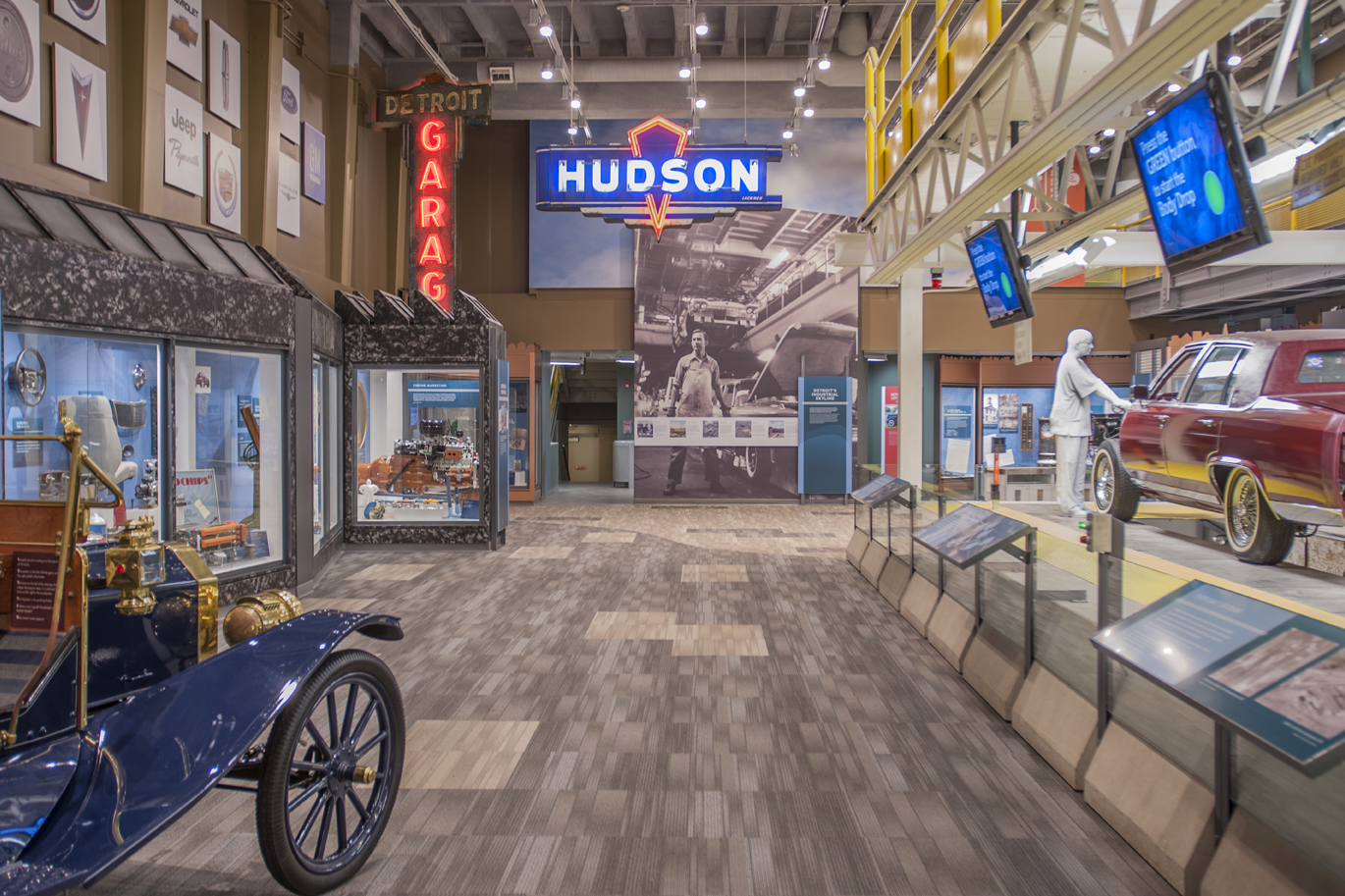The image captures the interior of an automotive museum, featuring a large, well-lit room with natural light. Prominently displayed on the left is a blue Model T car adorned with gold trim, and to its right, a burgundy red Monte Carlo style car with chrome spoke rims. Above the scene, two illuminated signs read "Hudson" in blue letters and "Detroit Garage" in bright red. A life-sized mannequin dressed entirely in white stands by the red car, as if about to open its door. The museum showcases various exhibits, including glass cases along the left wall containing a plethora of engine parts and historical information. Large TV screens hover over both cars, rotating through different displays, while informational plaques are placed below each vehicle. Additionally, a substantial black and white photograph in the backdrop depicts a man working on a car assembly line, adding a historical context to the setting.